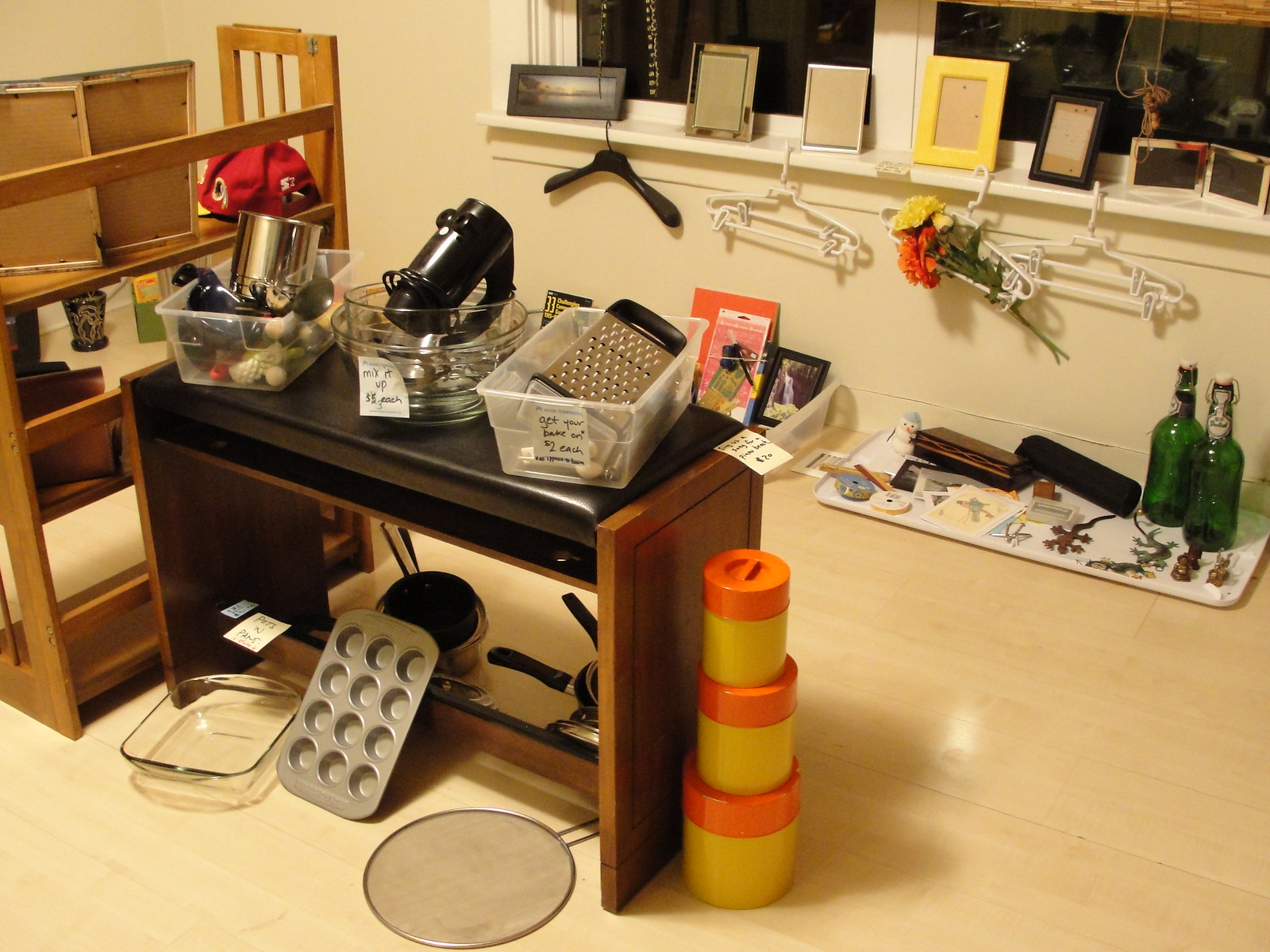The photo captures the cozy interior of a room being used for a garage sale. The room features a light, wooden floor and cream-colored walls, with natural light streaming in through a windowsill located in the back right. Various kitchen goods are meticulously organized throughout the space, occupying the floor, tables, seating, and even the windowsill.

In the center of the image, there is a black bench seat displaying several kitchen appliances in boxes. Each box has a Post-it note indicating the prices and some playful captions. One box, labeled "Get your bake on, $2 each," contains a cheese grater. Another, labeled "Mix it up, $5 each," holds a blender placed inside a bowl. To the left of these labeled boxes is an unmarked box containing a cupcake tin, a Pyrex bakeware dish, a strainer, and some jars and containers.

The background reveals additional items for sale, including food-grade fermentation bottles, hangers, and empty photo frames. Off to the left side, shelving units showcase a variety of other goods like cups and more photo frames. The assortment of items suggests that the seller is parting with many pieces from their kitchen collection. The overall atmosphere of the photo is inviting and well-organized, creating a pleasant browsing environment for potential buyers.